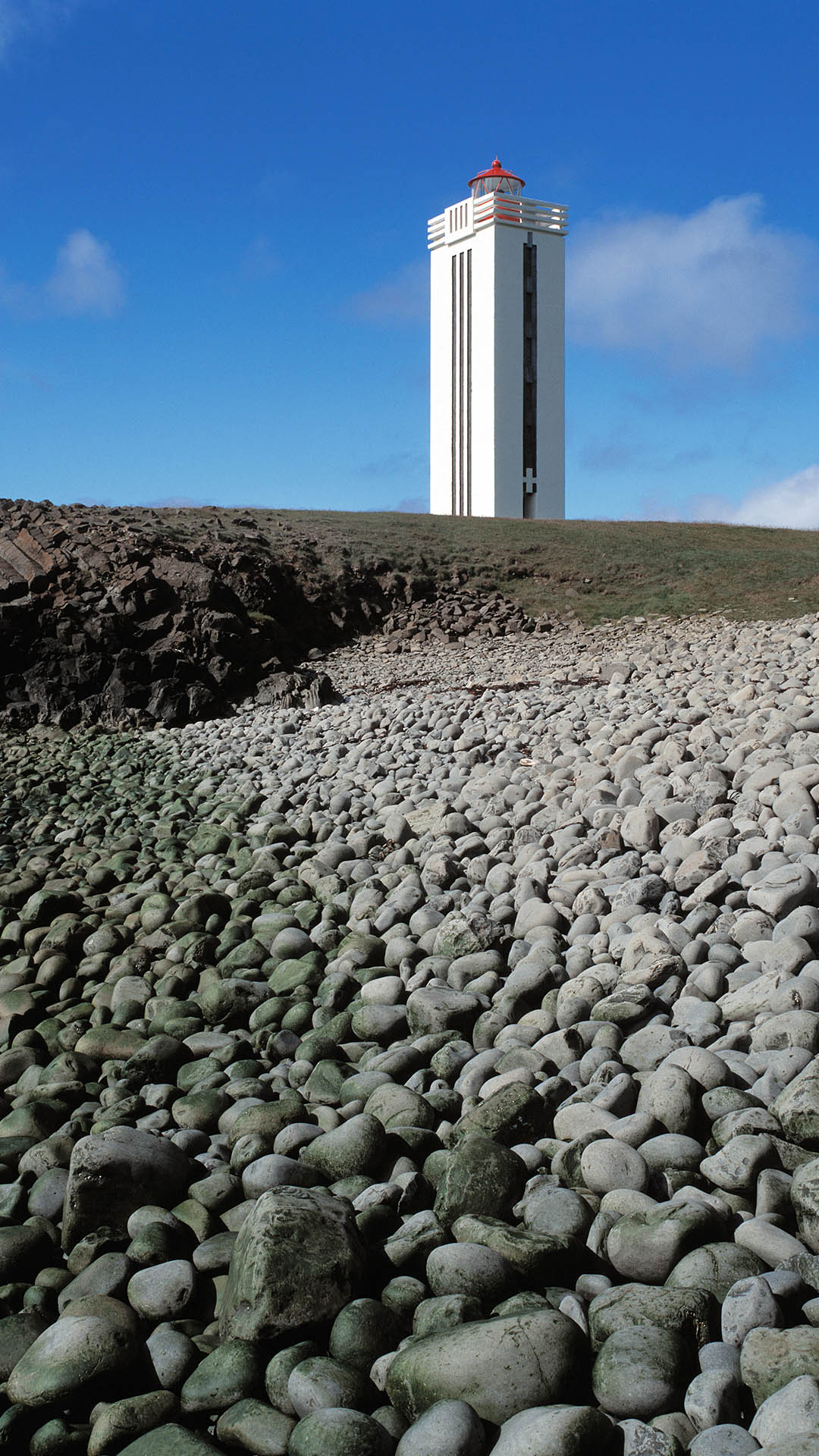This image features a tall, white, rectangular building standing prominently against a bright blue sky. The building, resembling a chapel or lighthouse, boasts black stripes on its sides and a white cross toward the bottom. At its apex, there's a dome with a red roof, encircled by a lookout platform adorned with white slots. 

The lower half of the image is dominated by a rugged landscape of large, gray rocks that vary in appearance: the rocks on the left side of the scene appear mossy and dark, as if wet, while those on the right look drier and clearer. The rocks transition into a middle section of brown-green grass and dirt, contributing to the earthy feel of the scene. The sky atop is largely clear, with a few wispy clouds overhead, providing a serene backdrop to the striking vertical structure.